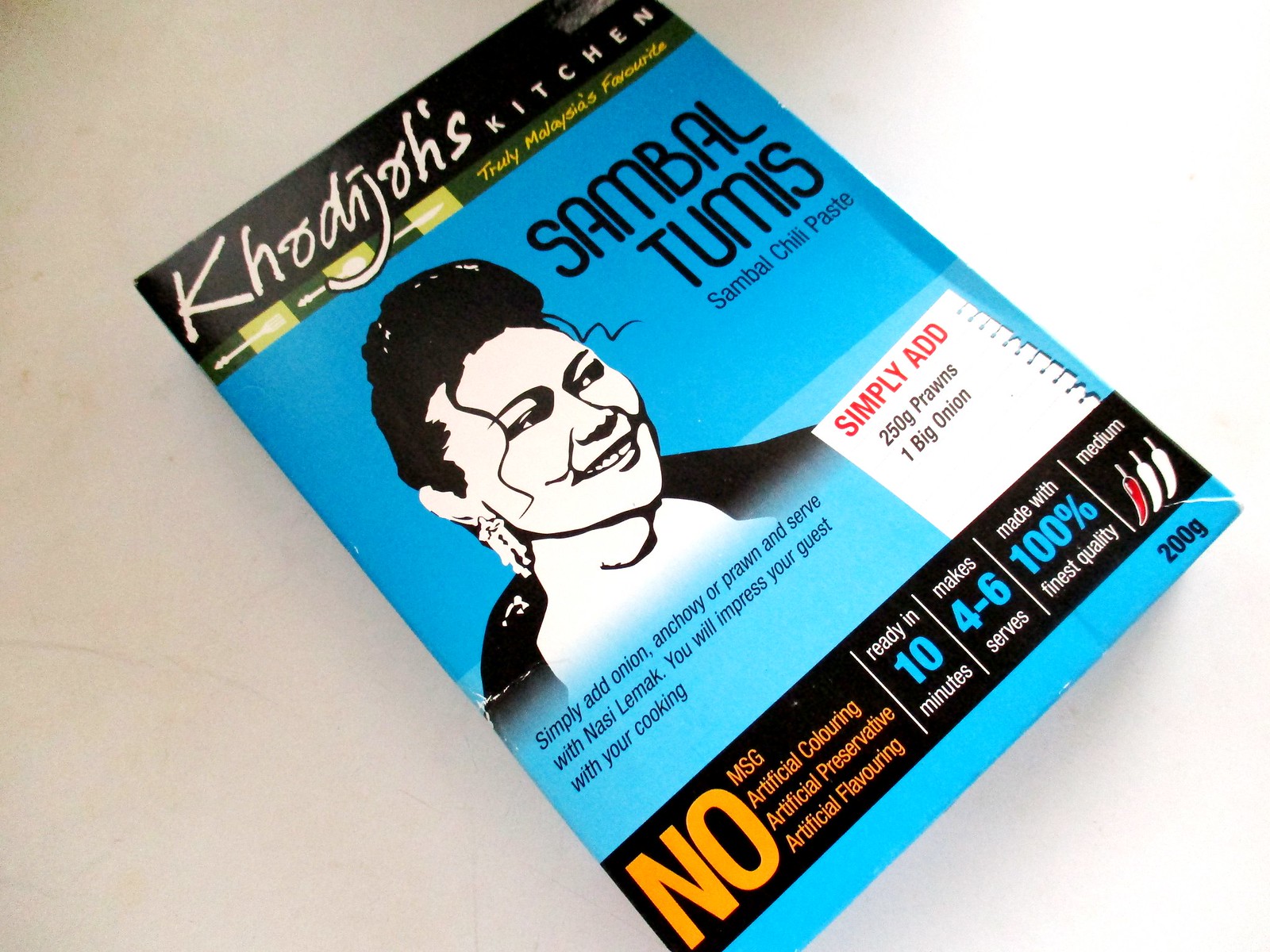This image features a packet of Sambal Tumis, a sambal chili paste from Kodijo's Kitchen, emblazoned with the tagline "Truly Malaysia's Favorite." The packet’s backdrop transitions from a deep blue at the top to a lighter blue towards the bottom. Dominating the design is a black-and-white image of a woman with a hair bun and long earrings, facing right. Instructions on the packet suggest that the chili paste can be enhanced by adding onions, anchovies, or prawns, and is ideal for serving with nasi lemak to impress guests. The packet specifies: "Simply add 250g prawns, one big onion." At the bottom of the package, it assures buyers of its premium quality with statements: "No MSG, no artificial coloring, no artificial preservatives, no artificial flavoring." It also notes the product’s preparation details: "Ready in 10 minutes, makes 4-6 servings." Additionally, it has a spice level indicated as medium, with one out of three chili peppers colored red. The packet weighs 200 grams.